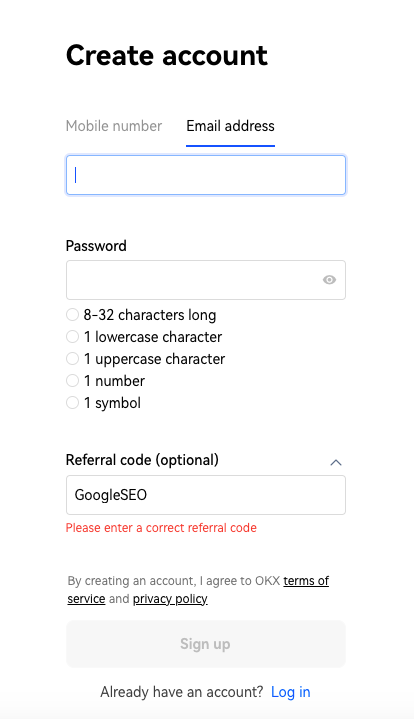"Screen Capture of OKX Account Creation Page: 

The image displays a login screen with a clean, white background and predominantly black font for optimal readability. At the top of the screen is the bold, black text ‘Create Account’. Below this, there are two sub-menus: 'Mobile Number', which is grayed out, and 'Email Address' underlined in blue. 

Further down, there is a blue box containing a blue cursor, followed by the black text 'Password' accompanied by a gray eye icon. This section also lists password criteria, each with a white circle beside it, including: 8 to 32 characters long, one lowercase character, one uppercase character, one number, and one symbol.

The next section contains the black text 'Referral Code (optional)' with a gray input box below it that displays ‘google seo’. Underneath, a red error message states, 'Please enter a correct referral code’.

Further down, gray and black text reads, 'By creating an account I agree to OKX Terms of Service and Privacy Policy,' with 'Terms of Service' and 'Privacy Policy' underlined in black. 

There is a 'Sign Up' button with a capitalized 'S' in 'Sign’. Below this, the black text reads, 'Already have an account?' followed by the blue text 'Login'. The bottom of the image features a thin, gray bar. Overall, the screen is designed to be clear, bold, and easy to read, catering well to the vision-impaired.”